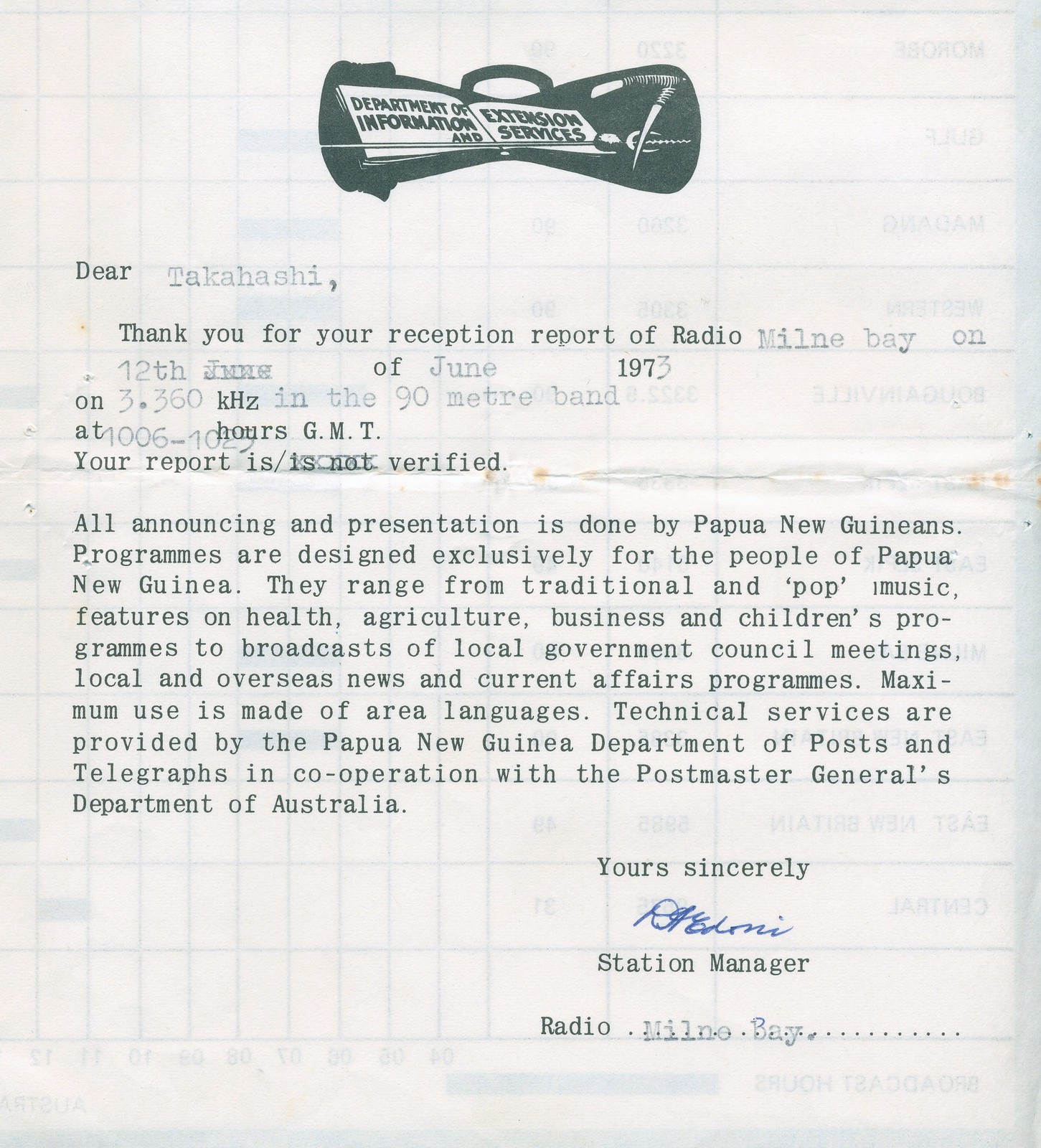This image features a typed letter printed on white paper with black and gray text, which has visible impressions of a grid from its back side. At the top center of the letter, there is a logo in dark blue-green color depicting a bag with a book inside, and the words "Department of Information and Extension Services" are written on the book in the same color. Below the logo, the letter begins with a formal typewriter font and is addressed as follows:

"Dear Takahashi, Thank you for your reception report of Radio Milne Bay on the 12th of June 1973, at 3.360 kHz in the 90-meter band at 1006/10 hours GMT. Your report is verified."

The letter continues to provide details about the radio station's programming:
"All announcing and presentation is done by Papua New Guineans. Programs are designed exclusively for the people of Papua New Guinea, ranging from traditional and pop music, features on health, agriculture, business, and children's programs, to broadcasts of local government council meetings, local and overseas news, and current affairs programs. Maximum use is made of area languages. Technical services are provided by the Papua New Guinea Department of Posts and Telegraphs in cooperation with the Postmaster General's Department of Australia."

The letter appears to be a template with various fields filled in using the same typewriter font, giving it a somewhat impersonal look. The signature at the lower right, written in blue ink, adds a personal touch and is signed by the station manager, though the signature itself is not legible.